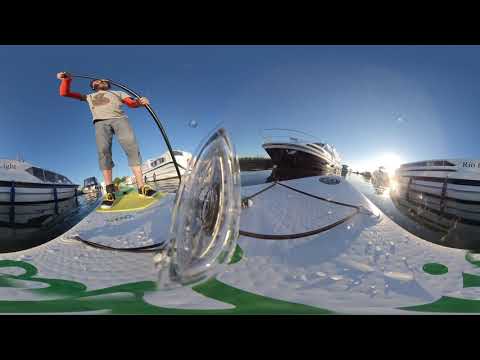The image captures a unique perspective from a low angle, possibly taken with a VR 360 camera, positioned on a white and green surfboard or paddleboard. The person standing on the board has their face obscured, wearing a white long-sleeved shirt, cut-off grayish-blue jeans, and black shoes, and is holding a curved paddle or pole, suggesting they are navigating water. The camera lens has created a slightly distorted, skewed effect, enhancing the scene's surreal quality. Surrounding the person, the bright blue sky meets a body of water populated by several large boats—one to the right, one to the left, and one directly behind—reflecting sunlight in a shimmering display. Additionally, the image features peculiar elements like a glassy, circular anomaly in the foreground and what appears to be icy, snow-like textures with some green patches, further adding to the image's intriguing and somewhat disorienting composition.